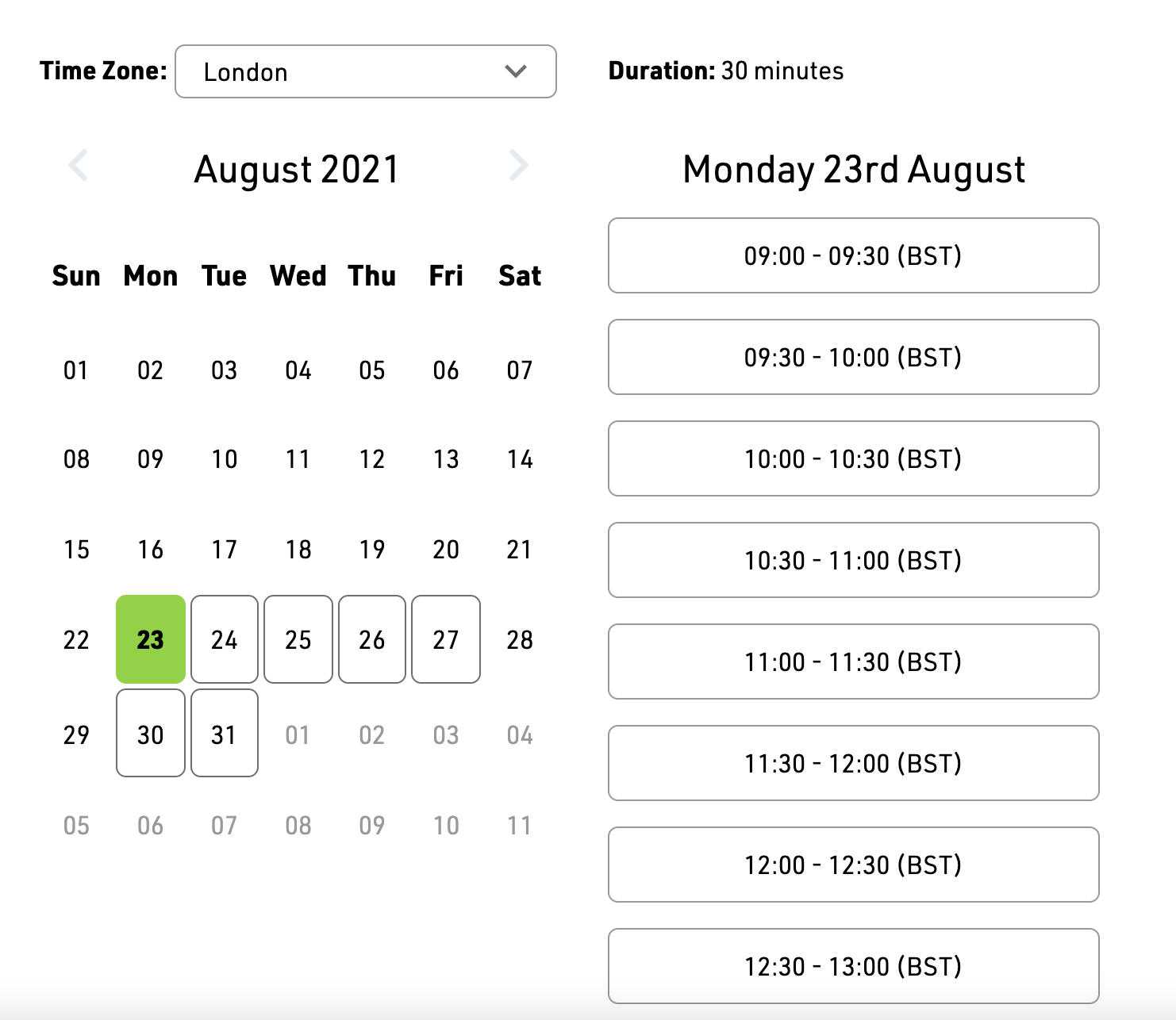The image features a user interface for scheduling or viewing appointments. Against a white background, the top section displays the label "Time Zone" followed by a dropdown box indicating "London" with a downward arrow for selection. Below, there is a field labeled "Duration: 30 minutes."

Centered in the interface, navigation arrows flank "August 2021," allowing the user to move between months. Beneath this, a calendar grid for August 2021 is displayed, where the 23rd is highlighted in green, signaling a special date or an active selection, and the dates from the 24th to the 31st are marked with blue squares.

On the right side of the image, the detailed schedule for Monday, August 23rd is listed. The schedule is divided into blue time blocks, each representing a 30-minute interval from 09:00 to 13:00 BST (British Summer Time). Specific time slots are as follows:

- 09:00 to 09:30 BST
- 09:30 to 10:00 BST
- 10:00 to 10:30 BST
- 10:30 to 11:00 BST
- 11:00 to 11:30 BST
- 11:30 to 12:00 BST
- 12:00 to 12:30 BST
- 12:30 to 13:00 BST

A light blue box runs across the bottom of the interface, perhaps acting as a summary or an additional option for user interaction. This detailed visual ensures easy navigation and clear visualization of time slots and selected dates.